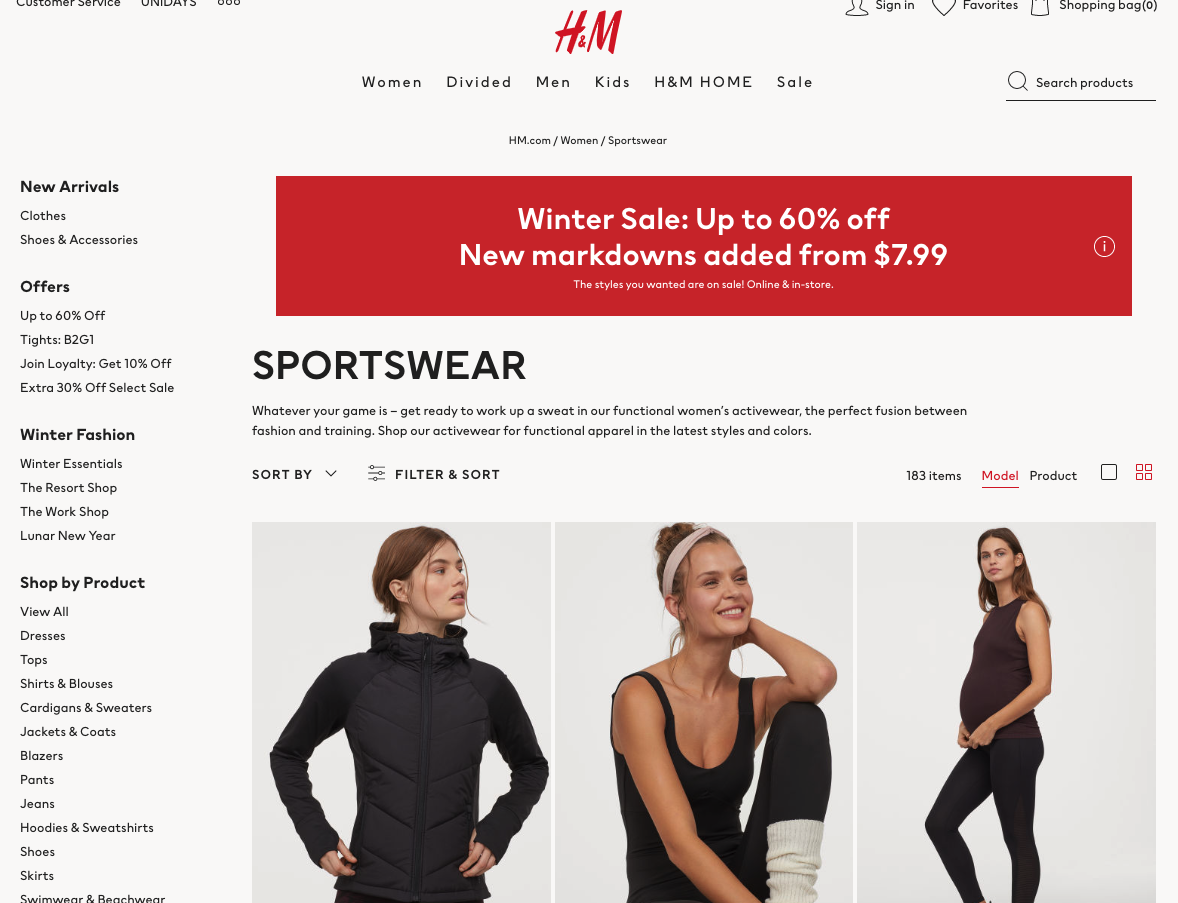This is a color screenshot from the H&M website. At the top, the H&M logo is displayed prominently in red letters. Below the logo, the main navigation menu includes categories such as Women, Divided, Men, Kids, H&M Home, Sale, and Search Products. 

On the left side of the screen, a vertical menu offers a comprehensive list of shopping categories and promotions, including New Arrivals, Clothes, Shoes and Accessories, Offers, Up to 60% Off, Tights B2G1, Join Loyalty, Get 10% Off, Extra 30% Off Select Sale, Winter Fashion, Winter Essentials, The Resort Shop, The Workshop, Lunar New Year, Shop by Product, View All, Dresses, Tops, Shirts and Blouses, Cardigans and Sweaters, Jackets and Coats, Blazers, Pants, Jeans, Hoodies and Sweatshirts, Shoes, Skirts, Swimwear and Beachwear.

To the right, a large red banner with white text announces the Winter Sale, offering discounts of up to 60% off. Beneath the banner, it reads, "New Markdowns Added from $7.99. The Styles You Wanted are on sale online and in store."

The main content area features three images of fair-skinned women in different activewear ensembles:

1. The first woman, with auburn hair pulled back with tendrils framing her face, looks to the right. She is wearing a fitted black jacket and has her hands on her hips.
   
2. The second woman, with her hair pinned up and a white headband, sits with her left knee raised and her left elbow resting on it. She is looking to the right and smiling. Her outfit includes a black tank top, black leggings, and white slouchy socks.
   
3. The final image shows a pregnant woman looking directly at the camera. She has dark, shoulder-length hair and is standing sideways. She is wearing a dark brown, short-sleeved top and tight black leggings.

Additionally, a subtext under the promotional banner encourages customers to shop their activewear collection described as the perfect blend of fashion and function, ensuring readiness for any workout with the latest styles and colors.